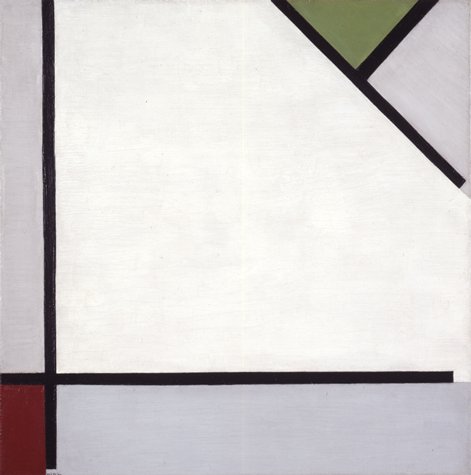The image is an abstract, esoteric piece of art featuring several intersecting black lines and distinct color sections. On the left side, there's a prominent vertical black line extending almost the entire height of the image, intersected near the bottom by a horizontal black line that creates a cross shape. This intersection forms a small box in the bottom left corner that is filled with a dark maroonish red color. The remaining border in the lower left is a light gray hue.

Occupying the upper right section of the image is a diagonal black line, which shapes the central area into what appears to be a large white triangle with truncated tips. Alongside this main section, there's another intersecting black line forming an inverted T-shape. This intersection produces two smaller triangles: one green and one white. The overall composition is minimalistic yet detailed, characterized by sharp lines and contrasting colors that evoke a modern, abstract aesthetic.